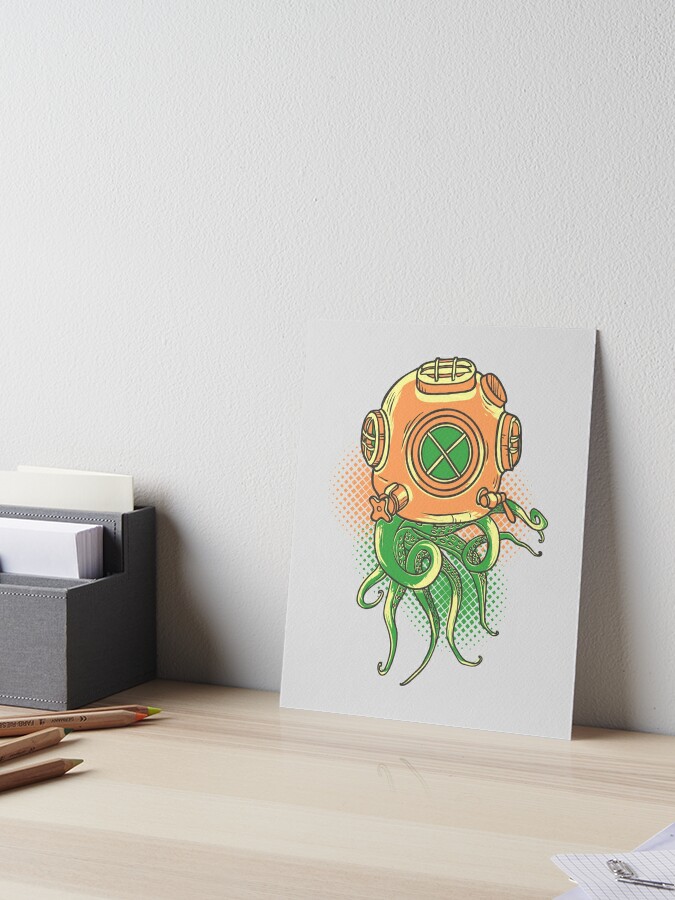The photograph captures a light wood grain desk surface adorned with various drawing items against a plain white wall backdrop. Dominating the scene, toward the center right, is a meticulously hand-drawn postcard-sized illustration of a whimsical green octopus, vibrantly detailed with a gradient from green to yellow towards its tentacle tips. This cartoonish octopus is donning an old-fashioned, large metal scuba diving helmet in shades of orange and yellow, featuring grates over its viewports and a turnable valve. On the lower left of the desk, several colored pencils lay scattered beside a gray organizer containing blank cardstock sheets, adding an artistic and dynamic element to the composition.